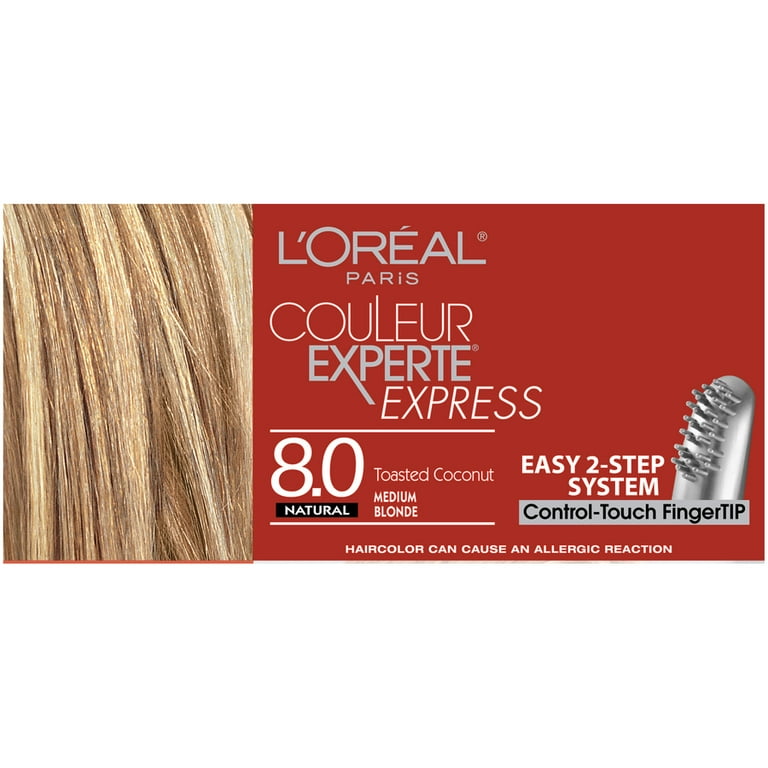This is a horizontal rectangular advertisement for L'Oreal Paris hair coloring. On the left third of the image, there is an example of streaky, multi-toned hair in shades of honey blonde and light brown. The right two-thirds of the background are a deep red-orange color. At the top, in silver text, it reads "L'Oreal Paris." Below that, in white and silver letters, it says "Couleur Expert Express." In between two thin white lines, it states "8.0 natural toasted coconut medium blonde." In the bottom right corner, white text declares, "Easy two-step system, control touch fingertip." This is accompanied by an image of a fingertip device with small nubs designed for easy application. At the very bottom, a disclaimer in white text warns, "Hair color can cause an allergic reaction."